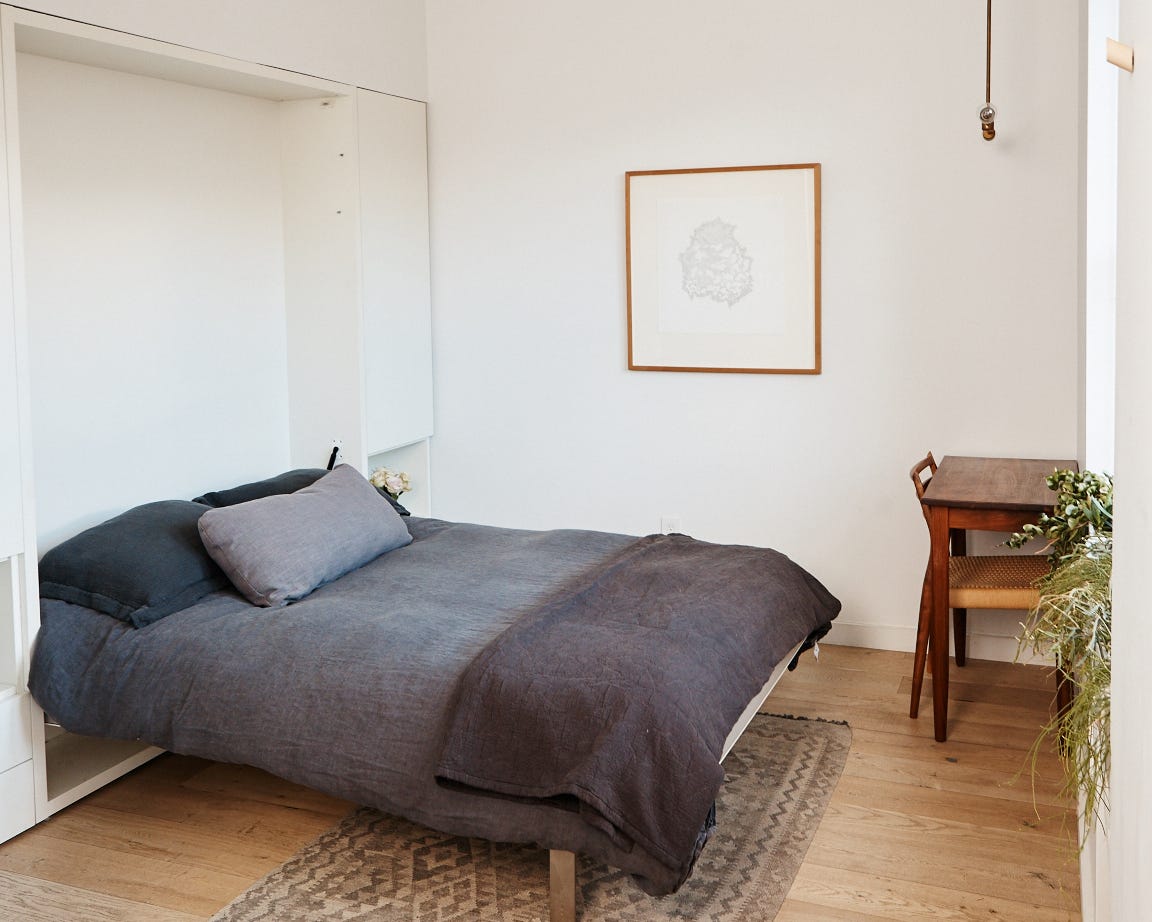This photograph captures a minimalist, Scandinavian-style bedroom with white walls. The focal point of the room is a Murphy bed, which is pulled down from the wall and features wooden legs that lift it slightly above the floor. The bed is dressed in various shades of gray linens with navy blue and gray pillows. Directly opposite the bed, a small wooden desk with a neatly tucked-in chair is illuminated by a single hanging light. A light wooden-framed print with a minimalist gray design hangs on the white wall above the bed. The light wooden floor adds warmth to the space, complemented by a geometric Turkish-patterned brown rug. Placed to the right of the bed, a windowsill holds vibrant green plants, enhancing the room's fresh and natural atmosphere. The subtle pops of color and the careful arrangement of functional elements harmoniously contribute to the room's serene ambiance.